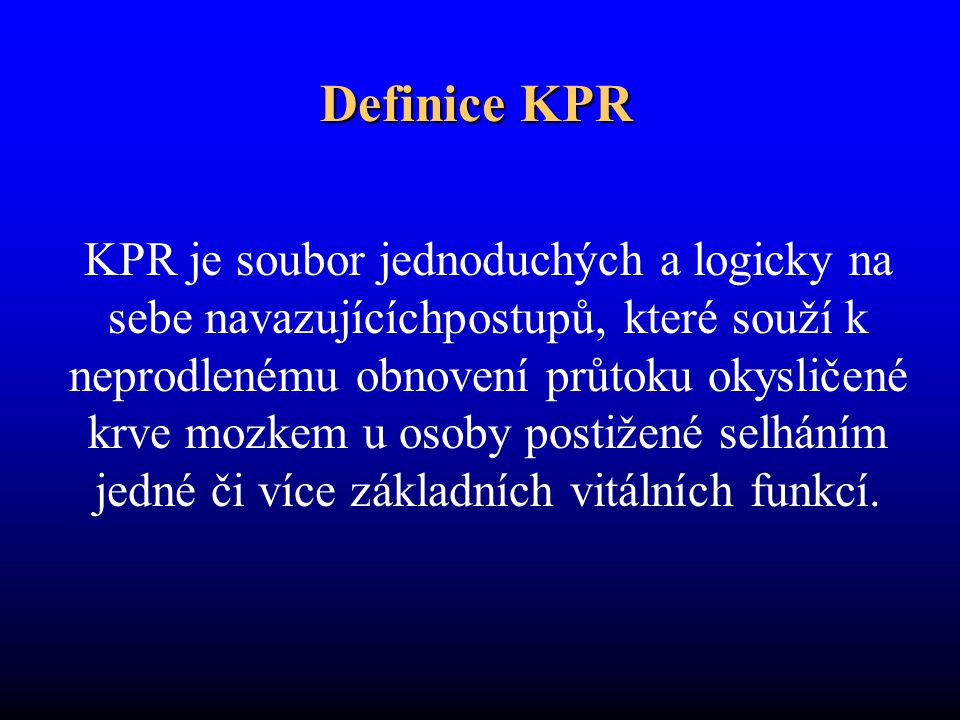The image is a horizontally oriented slide with a gradient blue background, transitioning from a vivid, bright blue at the top to a deep, almost black blue at the bottom. The text is in a non-English language and is written in Times New Roman font. At the top center, large and bold yellow block letters spell out "DEFINICE KPR". Below this, a long continuous sentence spans five lines of smaller white text, centered both horizontally and vertically. The text starts with "KPR" and is filled with accents, including little white circles above some 'u's and arcs above at least one 'z', suggesting the language might be from a Scandinavian country. The content appears organized, potentially resembling a learning or informational card.